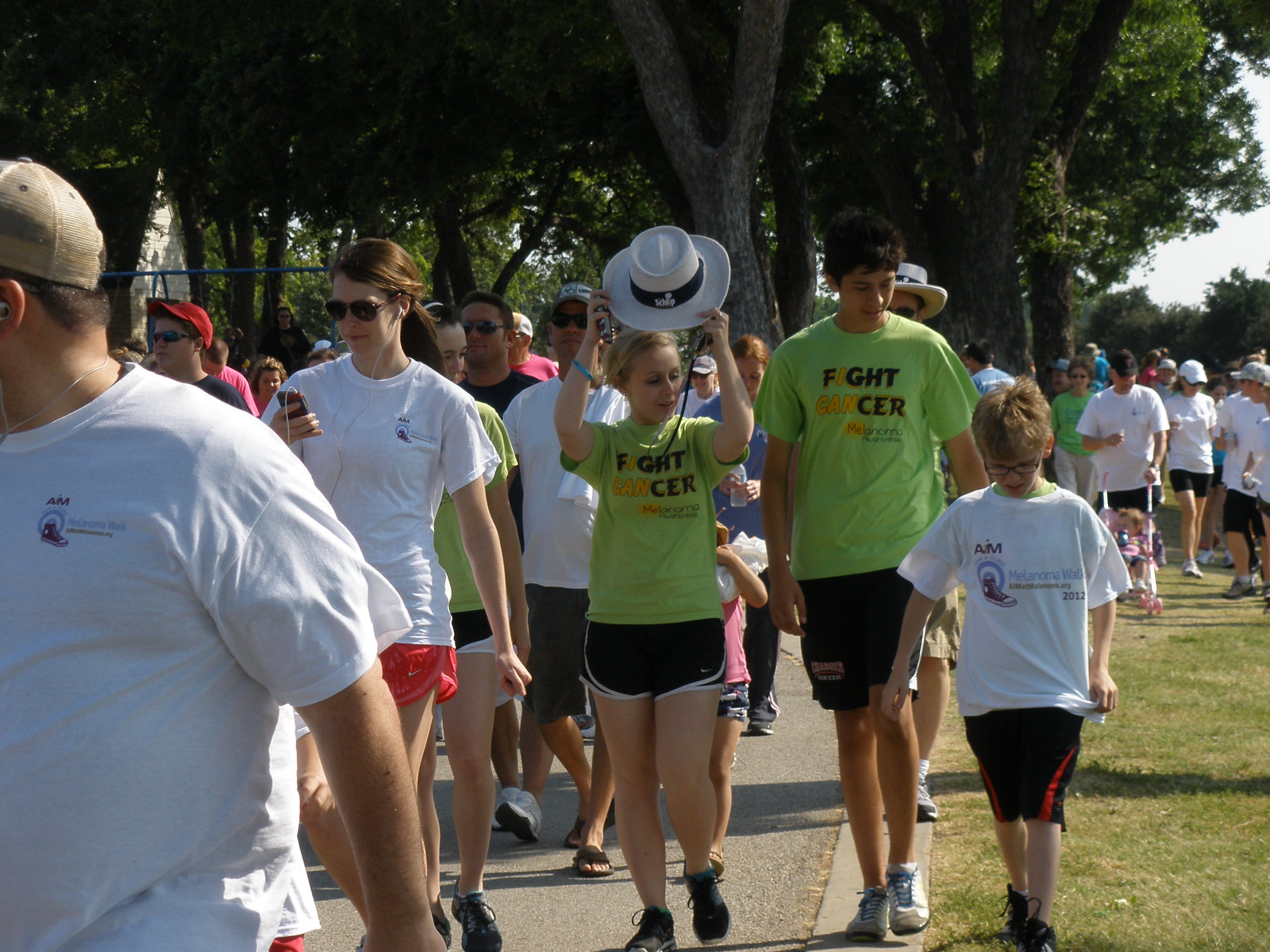This vibrant, sunlit photograph captures the bustling atmosphere of a charity walkathon or demonstration, likely focused on fighting cancer, given the green shirts with the message "Fight Cancer," where the "I" in "Fight" and "CAN" in "cancer" are highlighted in yellow, subtly conveying "I CAN." A mix of participants, predominantly clad in white shirts, are moving leisurely towards the camera, many wearing shorts, suggesting a warm summer day. The central figures include a teenage girl in a green "Fight Cancer" shirt, who is removing a white Panama hat with a blue band, and a taller teenage boy beside her, both looking down. To their right, a woman in a white shirt with sunglasses is engrossed in her phone. A younger child is seen on the bottom right in a white shirt with an indistinct logo, presumably from 2012. Large trees dot the area, casting long shadows over the paved path and grassy sections. The backdrop of foliage suggests a park setting, enhancing the picture's sense of community and purpose, as dozens flock together in a shared mission.